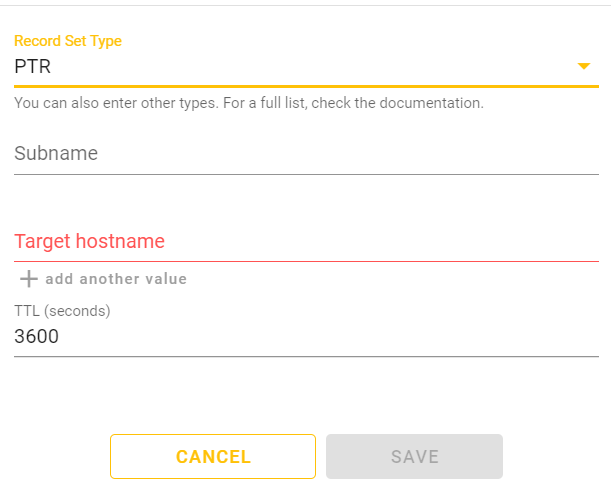The image depicts a settings menu for configuring record types, set against a white background. At the very top, a thin gray line stretches horizontally across the image. Immediately below this, aligned to the upper left corner, the phrase "Record Set Type" is displayed in yellow text. Directly underneath, the capital letters "PTR" are presented in black text. On the far right, a drop-down menu is noticeable, marked with a yellow directional arrow pointing downward.

Positioned beneath this is a prominent, thicker yellow line that extends horizontally. Below this line, in smaller black text, a message reads: "You can also enter other types. For a full list check the documentation." Following this message, there is a small space that leads into a section where bolder black text on the left reads "Sub Name." Below this, another thin black horizontal line appears.

Continuing downward, a space precedes red text on the left that states "Target Host Name," supported by another thin horizontal red line beneath it. Further down, charcoal gray text indicates "Plus Add Another Value," and beneath this, in all capitalized letters enclosed in parentheses, "TTL (Seconds)" is written. The number "3600" appears beneath, followed by a thin black line running horizontally.

At the bottom of the menu, two rectangular buttons are visible: the left rectangle features the word "Cancel" in yellow text, while the right rectangle displays "Save" in black text.